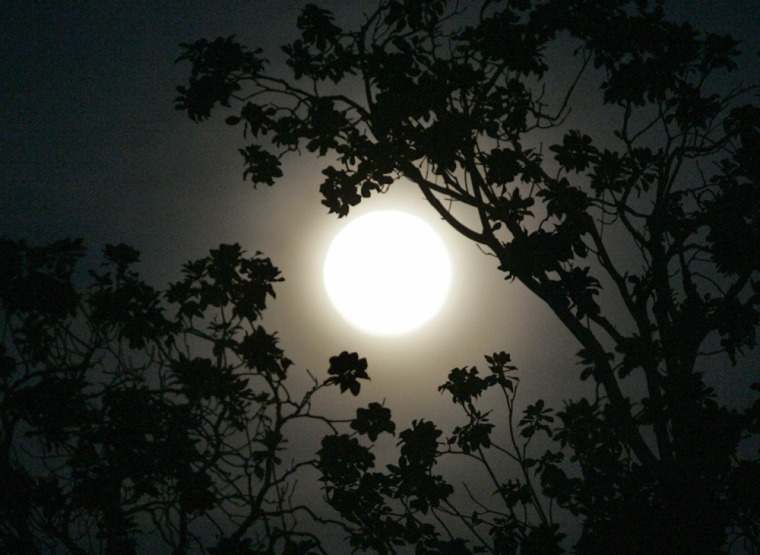This captivating nighttime photograph, rendered in striking black, white, and shades of gray, showcases a glowing full moon at the center of the image, casting a gentle glow across the dark sky. The textured details of the moon's surface are not visible, emphasizing its orb-like appearance. The photograph, possibly enhanced with filters and blurring for a dramatized effect, is framed by dense, silhouetted foliage that includes tree or shrub branches extending upward from the bottom of the image and arching from the right-hand side to the top. These clusters of leaves and branches, potentially resembling camellia flowers, create an intricate, natural border around the moon. With the lack of visible birds or additional textural details, the image focuses on the striking contrast between the moon's luminous glow and the dark, intricate silhouettes of the surrounding foliage.